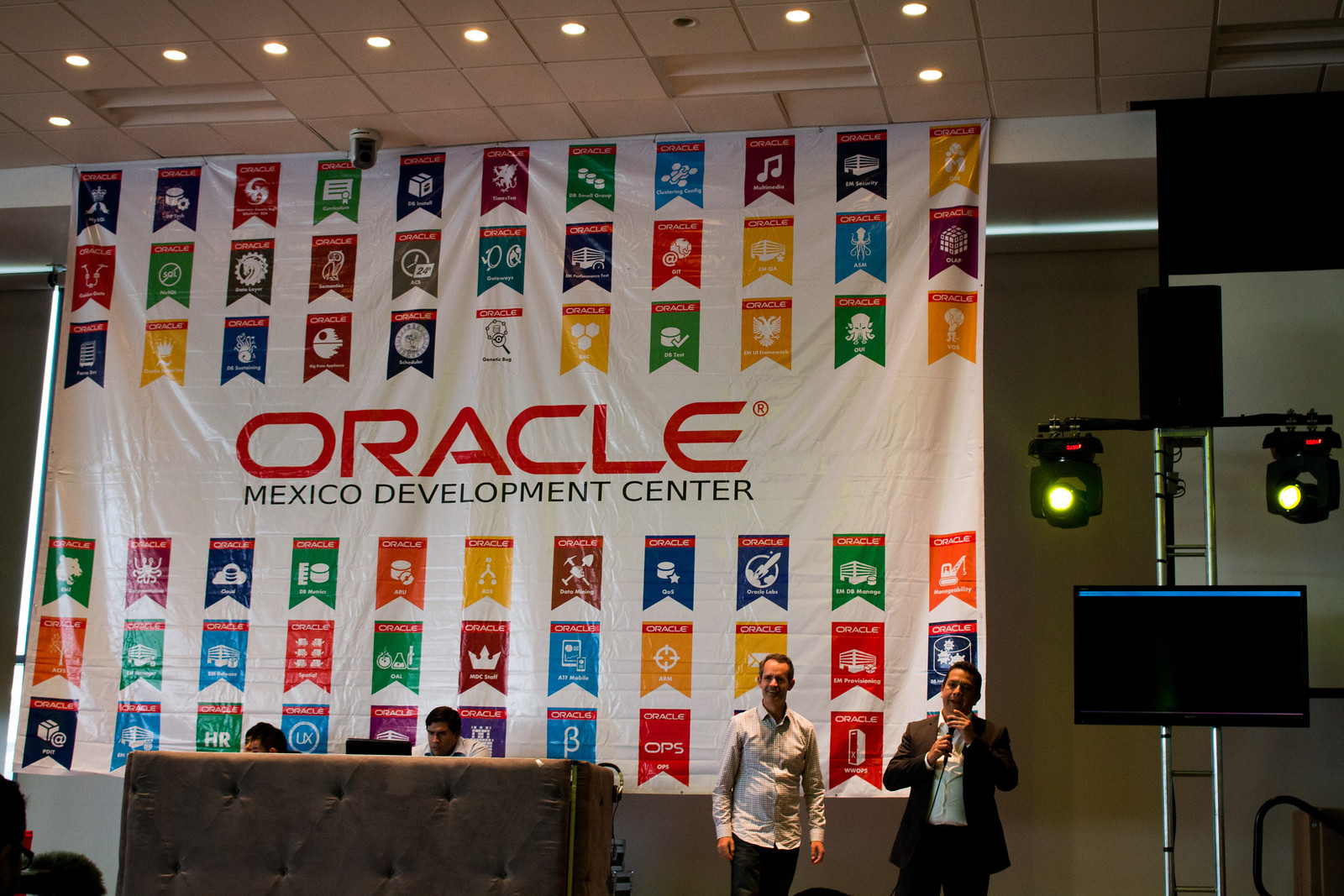The image captures a vibrant scene from a conference hosted by Oracle, titled "Oracle Mexico Development Center." The setting appears to be an indoor stage with a white backdrop adorned with a colorful array of Oracle logos in yellow, maroon, blue, green, orange, and pink. Prominently displayed in the center of the backdrop is the text "Oracle Mexico Development Center" in red letters. 

On the stage, towards the bottom right-hand side of the image, four men are present. Two of them are standing while the other two are seated. The man standing to the far right is dressed in a brown suit jacket, white collared shirt, and dark pants, holding a microphone as he addresses the audience. Beside him, another man is standing in a white long-sleeved shirt and dark trousers. The seated men are partially obscured behind a brown podium. 

The technological setup on the stage includes a flat-screen TV positioned to the right, equipped with overhead spotlights, and a black projector emitting a green light, suggesting an ongoing presentation. Additional stage lights and ceiling lights illuminate the scene, enhancing the overall visual dynamics of the conference setting.